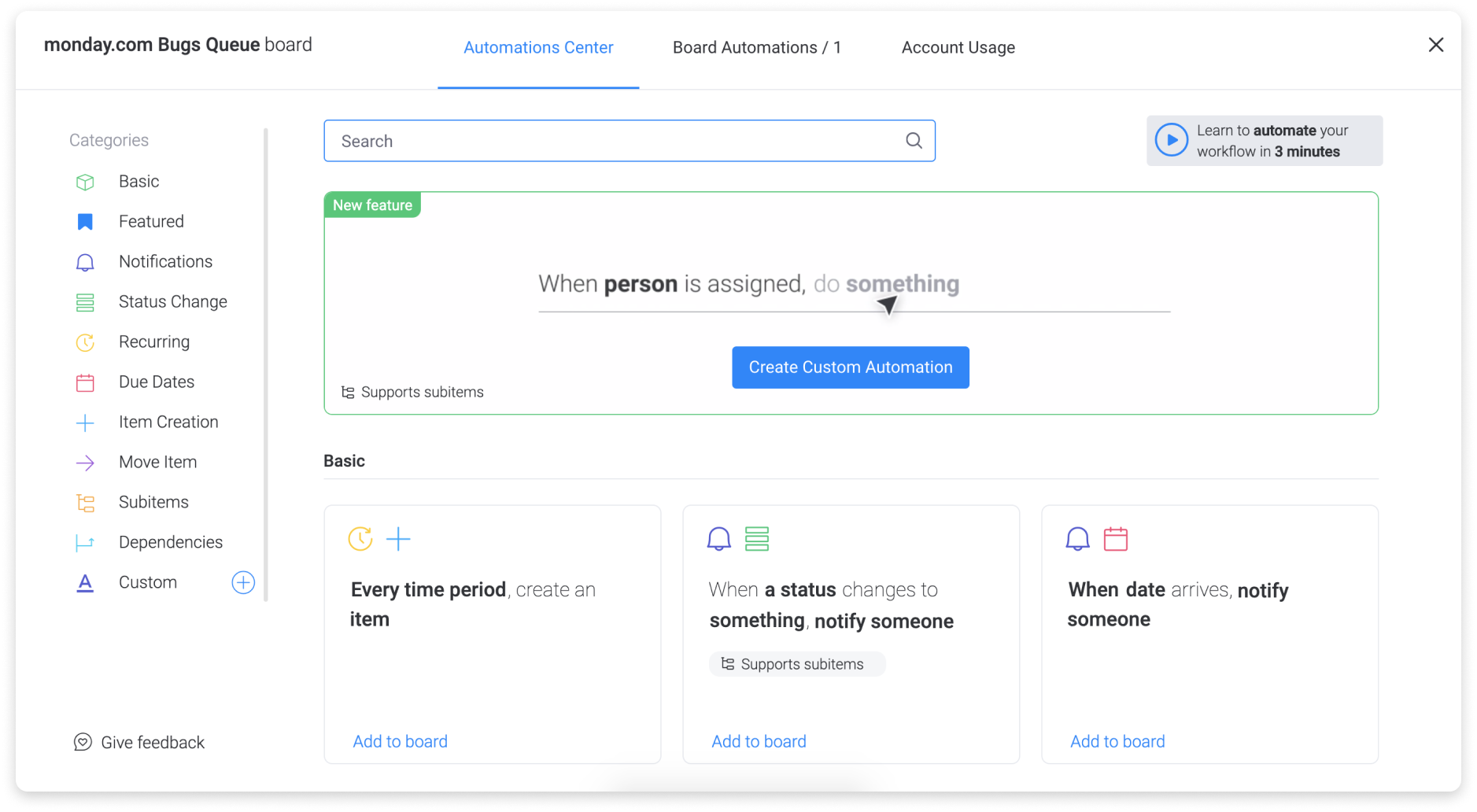The image depicts a section of the monday.com website, with a clear and detailed layout. In the top left corner, "monday.com" is prominently displayed in bold black font, followed by the word "Bugs" next to a cue board. 

Central to the image, the text "Automation Center" is underscored and highlighted in blue, emphasizing its importance. Adjacent to this label, it reads "Board Automations" followed by a forward slash and the numeral "1." Further to the right, "Account Usage" is mentioned with a notable "X" on the far right side of the screen.

On the left-hand side, there appears to be a list of categories: Basics, Featured, Notifications, Status Change, Recurring, Due Dates, Item Creation, Move Item, Sub Items, Dependencies, and Custom. Each of these categories is paired with corresponding icons that visually represent their functions.

Near the center of the interface, there is a search box labeled "Search," accompanied by a magnifying glass icon on its right side. Further to the right of the search box, text promotes learning to automate workflows in three minutes, indicating a user-friendly tutorial.

Below this section, there is a box highlighting new features, specifically "When person is assigned," along with an arrow indicating "Do something," leading to a "Create custom automation" button.

At the bottom of the image, three squares are presented. These are associated with different conditions, such as "Every time period in relation to status" and "When the date arrives, notify someone." Each of these squares includes an "Add to Board" option located at the bottom left of each square, suggesting actions that can be taken directly from this interface.